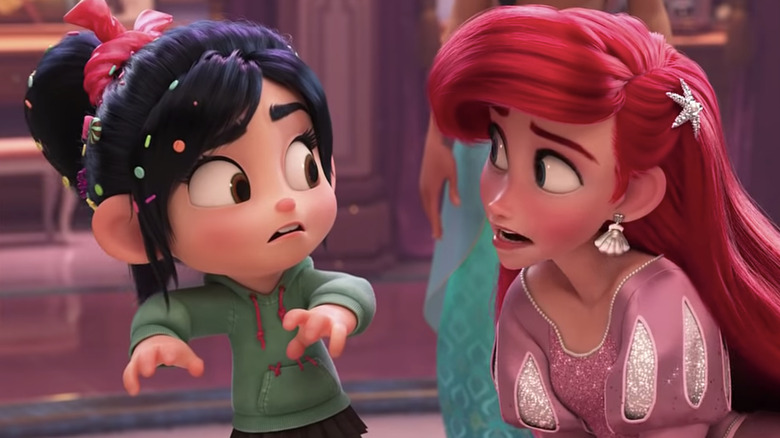In this vibrant, professionally animated scene, we are introduced to a regal character with striking long red hair adorned with a silver starfish decoration. Her stunning greenish eyes and red eyebrows complement her other accessories, including silver seashell earrings. She is elegantly dressed in a gown that combines shades of pink, white, and silver, exuding a royal aura that suggests she is a princess.

Standing behind her, partially visible, is another character clothed in a teal skirt, hinting at a continued palette of oceanic tones within the image.

Next to the red-haired princess is a charming little girl with her black hair styled in an updo, accentuated by a noticeable pink bow. Her hair is sprinkled with multicolored confetti or sprinkles in shades of green, teal, purple, and orange, giving her a whimsical appearance. Additionally, she sports a green and purple peppermint decoration in her hair. Her expressive brown eyes are framed by thick black eyelashes and eyebrows, lending an innocent and curious look to her face. This little girl is comfortably dressed in a seafoam-colored hoodie with pink strings, paired with a black skirt, creating a playful yet cohesive outfit that matches the overall aesthetic of the scene.